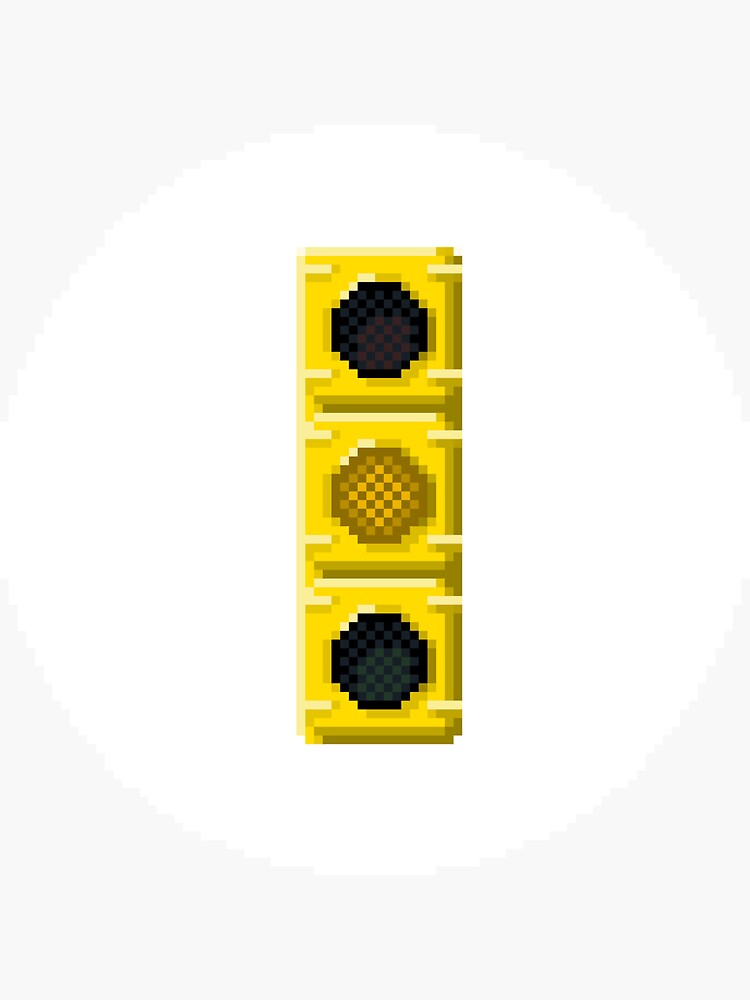This is a highly pixelated, 16-bit animated image of a yellow traffic light set against a vertical light gray rectangle border. At the center of this border, there's a white circle containing the traffic light. The traffic light depicts the typical arrangement of red, yellow, and green lights, although their colors are quite muted and less vibrant. The red light is at the top, the yellow light in the middle, and the green light is at the bottom, all embedded in a yellow light fixture with lighter yellow accents. This image resembles graphics found in classic Super Nintendo or Sega Genesis games, with a 16-bit sprite-like quality typical of retro gaming aesthetics.